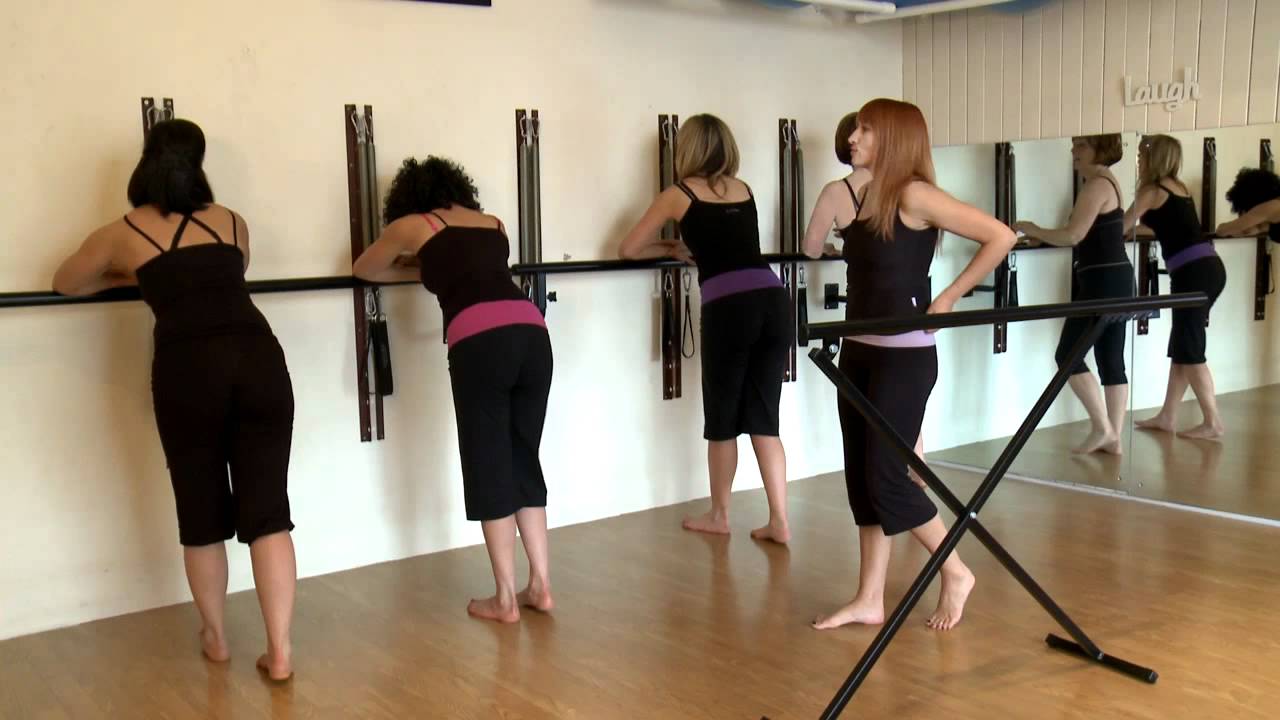In this indoor photograph, a group of five women occupies a room that resembles a ballet or dance studio, featuring white walls and a hardwood floor. Four women are aligned against a wooden barre attached to the wall, with their backs turned to the camera and their arms resting down at their sides. They are uniformly dressed in black clothing, which ranges from capris and camisoles to jumpsuits and skirts. Among these women, one has black curly hair, another has straight black hair tied in a ponytail, a third has blonde hair, and the fourth has red hair.

In the background, a fifth woman with long reddish-brown hair and wearing a black camisole and pants — also barefoot like the others — is walking closer to the photographer, with one hand on her hip, possibly engaging in conversation with the women against the barre. There is a shelf made of dark wood on the wall behind them. The right side of the room features a large mirror with the word "laugh" written on it. A metallic foldable stand with a rod is also visible in the room, contributing to the studio's functional setup. The overall scene suggests a tranquil moment in a dance or yoga class.